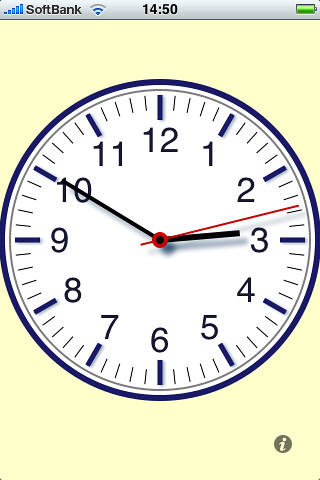This detailed illustration captures a screenshot from a mobile device, displaying a digital clock app on a yellow background. The clock itself features a simple round design with a white face, outlined in black, and marked with black numbers from 1 to 12. The current time displayed is 2:50, indicated by traditional black hour and minute hands, along with a red second hand. At the top of the screenshot, icons show a fully green battery, Wi-Fi connectivity, SoftBank signal strength, and the time 14:50 in military format, confirming the screenshot was taken from a cell phone. This comprehensive depiction combines elements of an analog-looking graphic clock within a digital interface.